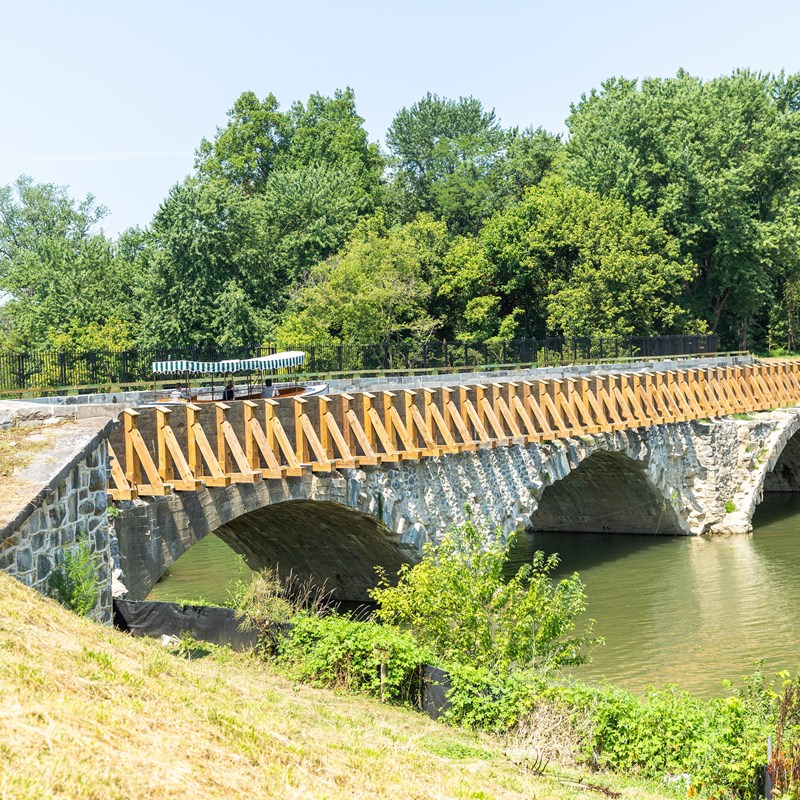The photograph depicts a scenic stone bridge with a triple arch design, gracefully spanning a river with a greenish tint. The image is taken from the left-hand side, offering a view across to the right-hand side of the bridge. In the foreground, a grassy hill descends towards the riverbank. The bridge, constructed from intricately carved stone in various shades of grey and accented with thick white grout, features distinctive triangular wooden beams along its sides, providing structural support. 

On the bridge, towards the left end, a boat with a green and white striped awning is visible, carrying three passengers seated under the shade of the awning. The surrounding environment is lush with tall, leafy trees behind the bridge, adding to the natural beauty of the scene. The river beneath the arches flows calmly, bordered on one side by a low stone wall intertwined with vegetation that may include ivy or blackberry bushes, possibly reinforced with black landscape cloth for erosion control. Above, the sky is partly cloudy, enhancing the serene atmosphere of this picturesque setting.